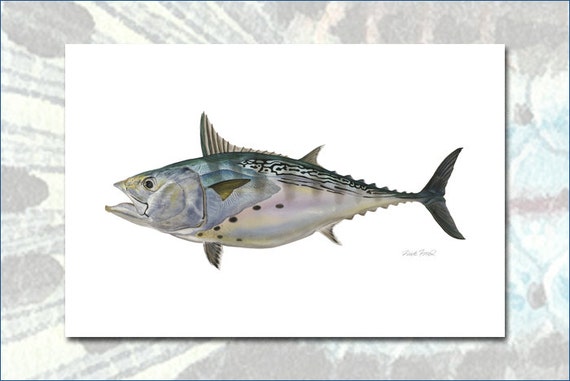The image features a detailed drawing of a large fish, facing left with its tail on the right. The fish has a silvery belly that transitions to a bluish hue toward the top. Its head and neck exhibit a shiny blue-purple color with a purple glow around the gill area. The dorsal side has black wavy stripes extending from the back of the head to the tail, and the body is adorned with small brown dots. The fish has a prominent mouth and a variety of fins: a large dark green one on top in the front, a smaller fin at the back on top, and two tiny fins on the belly—one near the front and one near the back. Its tail features two fins, one pointing up and one down. The fish is set against a plain white background with a marble-textured border and a thin blue line framing the entire image. Additionally, small wordings at the bottom right corner identify the species’ name.